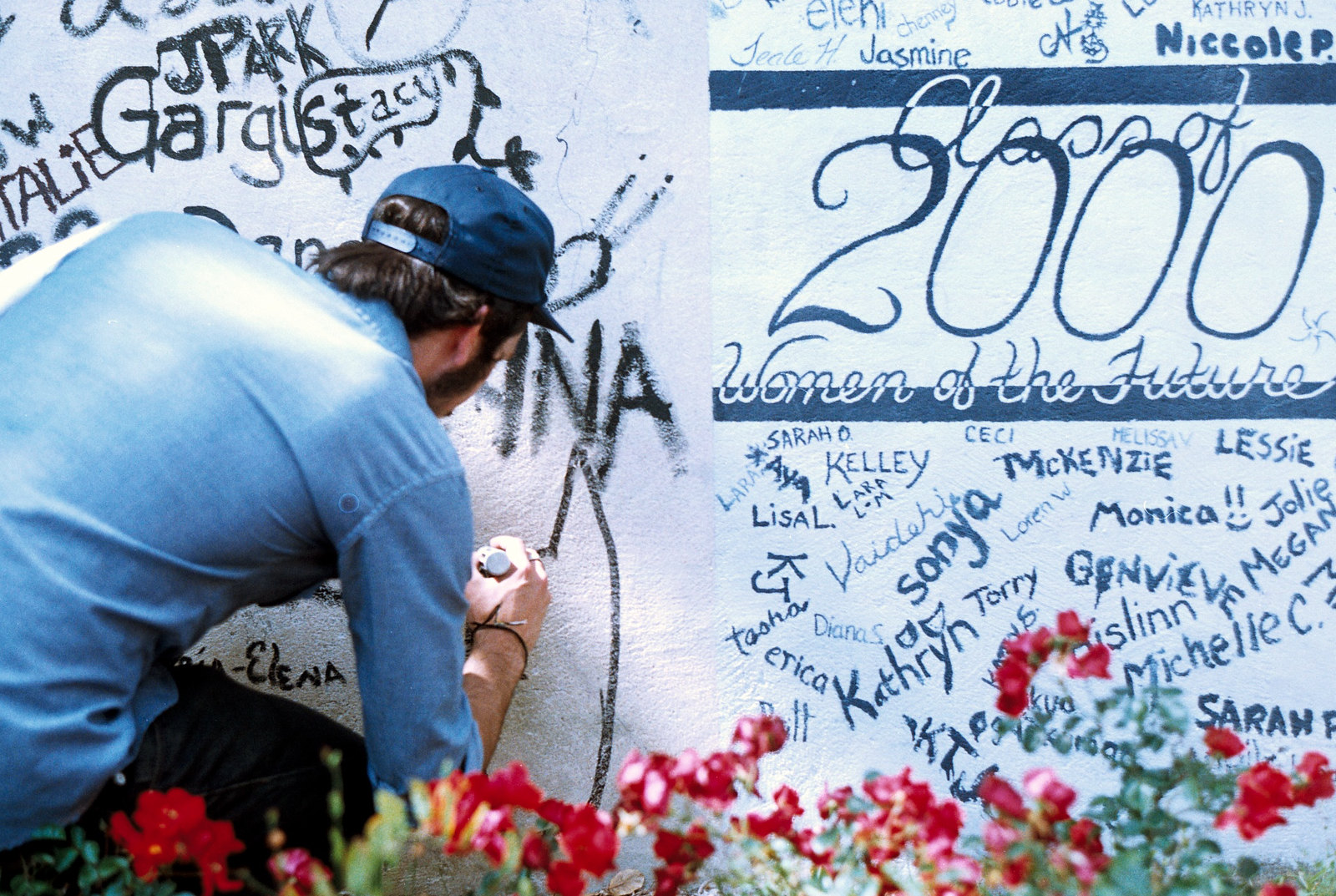In the foreground of the image, an array of red flowers with green stems stretches across the bottom, slightly blurred. The focal point reveals a man on the left-hand side, engrossed in graffitiing a wall with a thick black marker. He's dressed in a long-sleeved denim shirt, a darker blue baseball hat, and black pants, with brown hair visible under the hat. The wall he is adorning is painted in two distinct sections: the left side in white and the right side in an ivory white shade.

The ivory white section on the right prominently displays the title "Class of 2000, Women of the Future" in a professional font, surrounded by several names, each inscribed differently. On the white section to the left, multiple names written in black can be seen, and the artist is currently adding an illustration of an eared creature. The scene appears to be outdoors, likely in the vicinity of a school, capturing a moment of artistic expression in the middle of the day.